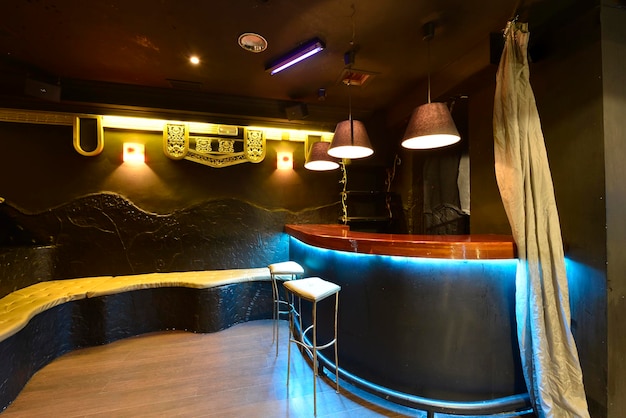The image captures an empty, professional-quality photograph of a small, possibly basement bar. Dominating the right side of the image is the main bar area with a sleek, shiny brown wooden countertop. Beneath this countertop, blue lighting adds a glowing effect, enhancing the modern ambiance. Above, three brown round lampshades hang from the ceiling, casting light onto the bar. In front of the bar, two white backless stools with silver frames stand ready for use.

To the left, a continuous white wavy bench with a three-dimensional design is set against a dark gray, curvy wall. This wall features two sconces, adding a subtle touch of light. Near the bar is a white curtain, possibly intended to cover the bar area.

The floor is made of light brown wooden laminate, providing a warm contrast to the darker elements. The ceiling is a deep gray, adorned with a blue purplish-black light tube, adding a futuristic element. The entire scene is devoid of people, alcohol, or any activity, creating a stark yet stylish atmosphere. The color palette includes black, white, brown, yellow, and blue, contributing to the overall modern and sophisticated feel of the space.